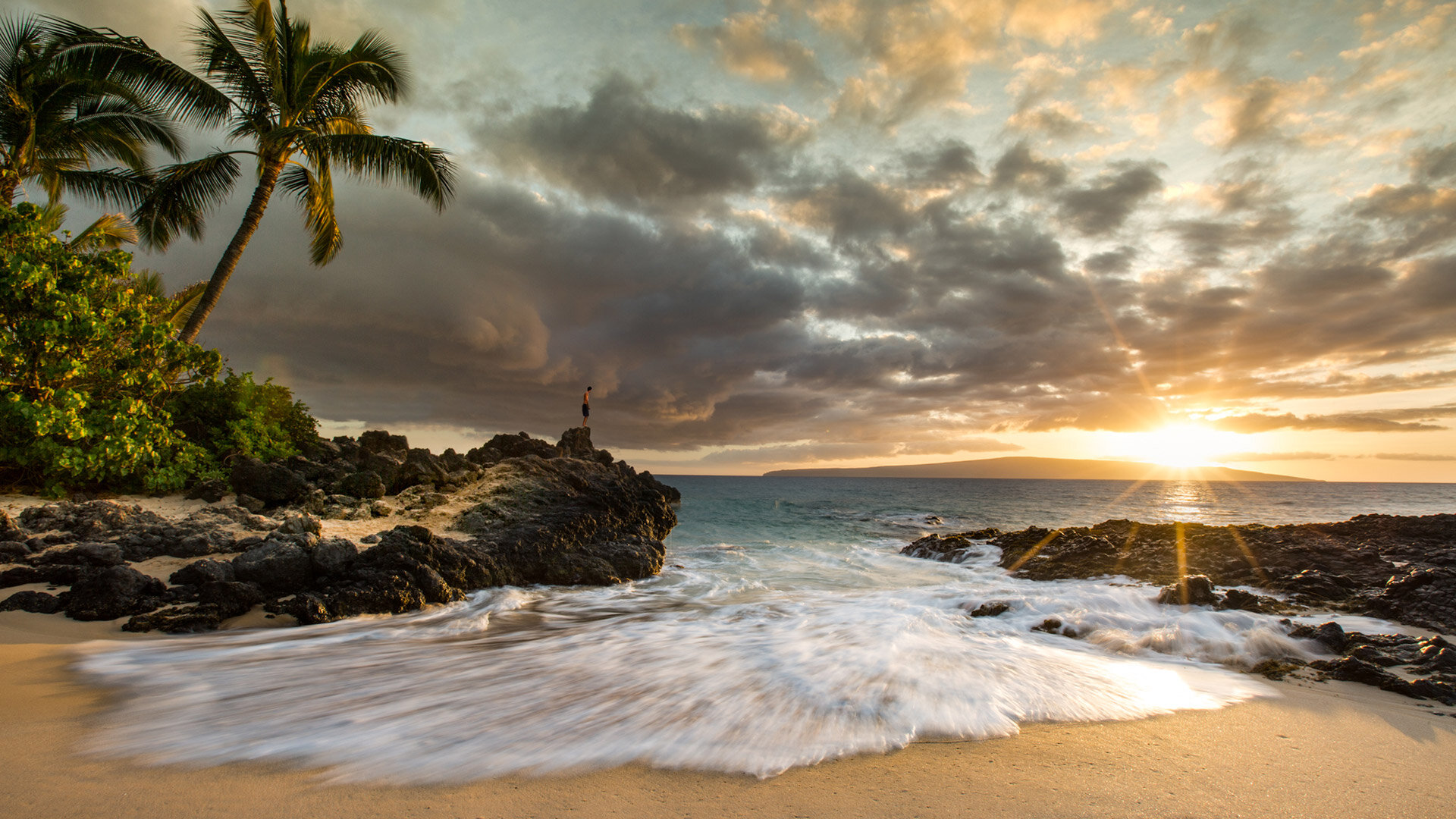A breathtaking landscape image captures a serene yet dramatic scene at a tropical beach. The photograph, a work of digital art utilizing long exposure, showcases the water rolling onto the sandy shore, creating a feathered, ghostly effect. Central to the view is a rugged outcropping of rocks upon which a thin, light-skinned man with dark shorts and black hair stands, gazing thoughtfully at the expansive ocean. To the left, swaying palm trees and lush green bushes adorned with yellow flowers sit against an increasingly stormy backdrop.

The sky is filled with dark gray, menacing clouds hinting at an approaching storm, yet, near the upper center-right of the image, the rays of the setting or rising sun pierce through, casting a bright, ethereal glow. Beyond the shoreline, where the turquoise waves crash into the island, the ocean turns frothy white as it meets the sand. The stunning, idyllic scene balances the tranquil beauty of a tropical paradise with the impending drama of a storm, making for a simultaneously peaceful and dynamic composition.